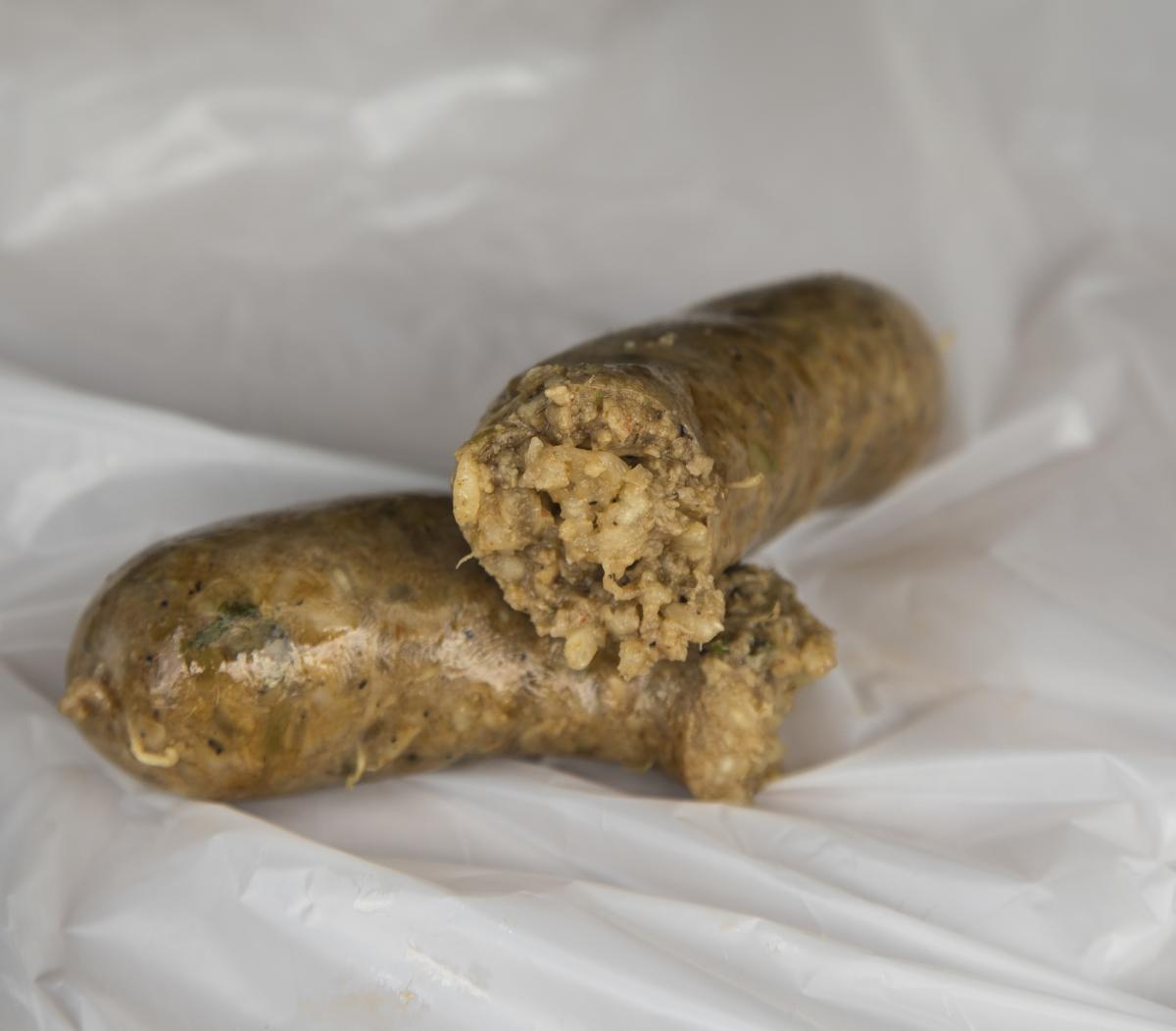In this close-up, high-quality image, two browned sausages are displayed atop a crinkled, white piece of plastic, which could be a garbage bag. The sausages are cut in half, exposing their juicy interiors filled with ground meat and an array of herbs and spices, including visible black pepper and green dried herbs. The sausages have a slimy, greasy sheen on their casings, and one of them has a short white string attached at the end, likely from the manufacturing process. They are arranged with one sausage lying horizontally at the bottom, while the other lays vertically over it. The plastic surface beneath them is wrinkled and features shadowed areas, enhancing the texture of the image.